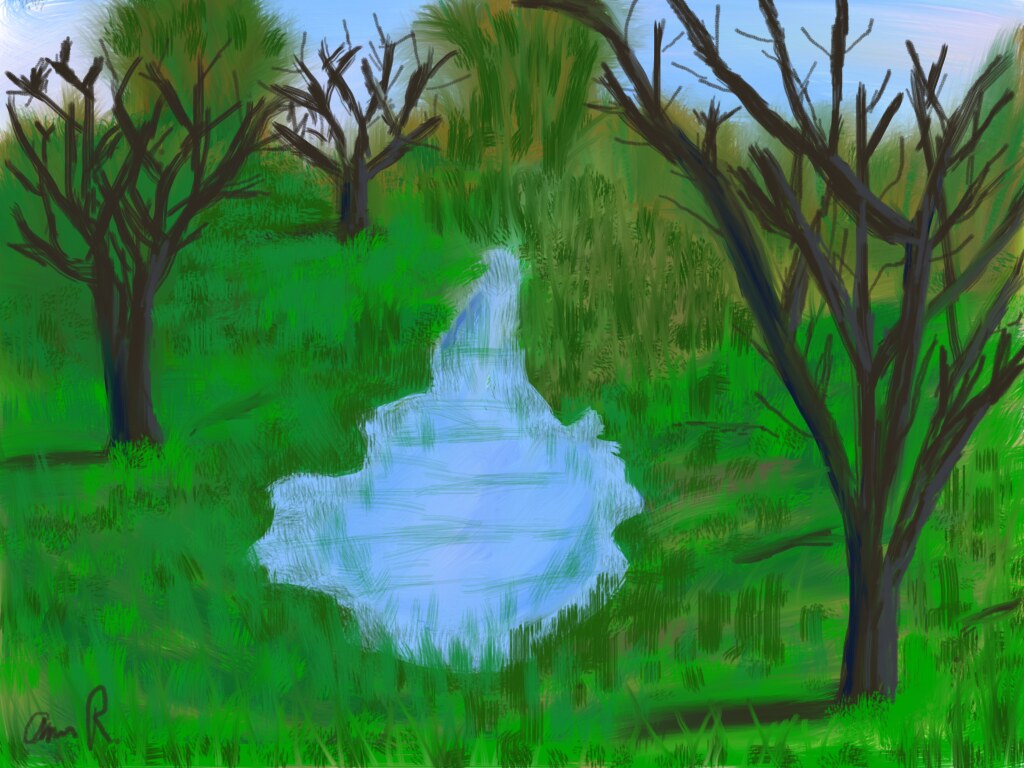The painting depicts a serene forest landscape with a mixture of barren brown trees and vibrant green grass and shrubbery. Some trees are sparse and leafless, suggesting a winter or early spring setting, while other foliage remains lush and verdant. Central to the composition is a bulbous-shaped pond, light blue in color, reflecting the sky and wispy white clouds above. The sky itself is a soft hue of light blue, enhancing the tranquil atmosphere. Shadows from the trees cast onto the grass provide depth and perspective. The artist, identified as Omen R., has signed their name in the bottom left corner of the artwork. The medium used appears to be watercolor, lending a delicate and ethereal quality to the scene.